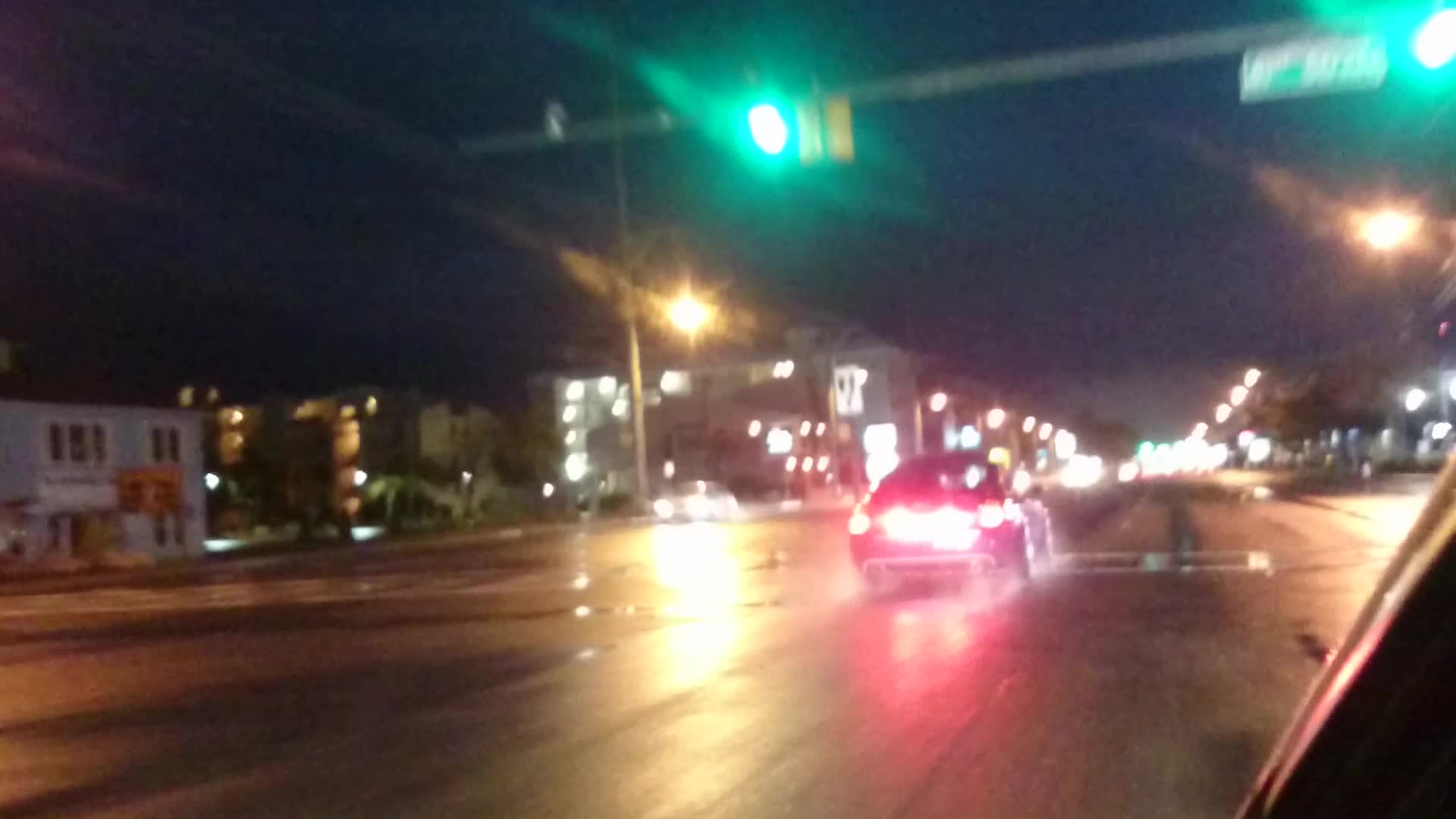A blurry nighttime street scene captures the view from inside a car looking out through a side window. The focus is on an intersection with American-style traffic lights suspended above the road. The green light is just visible, suggesting it has recently changed. A car is ahead, its red brake lights illuminated against the slick, damp road. Across the intersection, headlights of an oncoming vehicle add to the ambient glow. Building lights dot the background, and a few low-rise buildings, varying from two to four stories, are discernible. The street sign on the traffic light arm is indistinguishable due to the blur. The image conveys a damp, dark atmosphere, with reflections from various street and building lights enhancing the scene's nighttime setting.